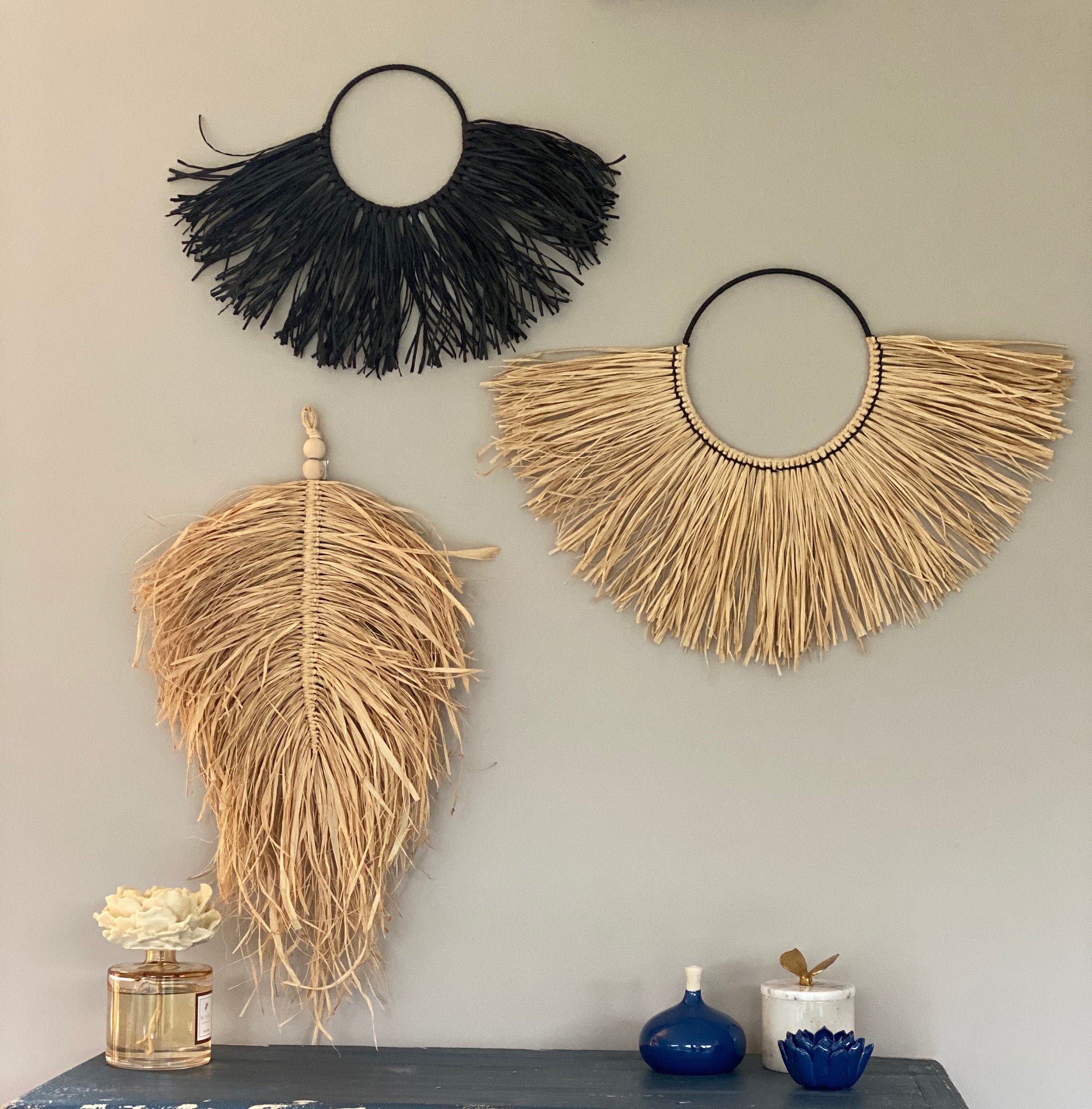The indoor color photograph features a cream-colored wall adorned with three distinct wall hangings made from natural materials, primarily straw and bamboo. Two of the wall hangings have a circular design with fanned-out bamboo strands, while the third features a more triangular or feather-like shape, braided from rattan. Below the wall art is a side table with a distressed dark gray paint job. On this table sits an old perfume bottle filled with flowers, a blue jar with a white stopper, a bowl shaped like a succulent, and a white jar with a gold handle. The ensemble of items on the table and the intricate handmade wall hangings suggest that the image may be intended to advertise these decorative pieces.